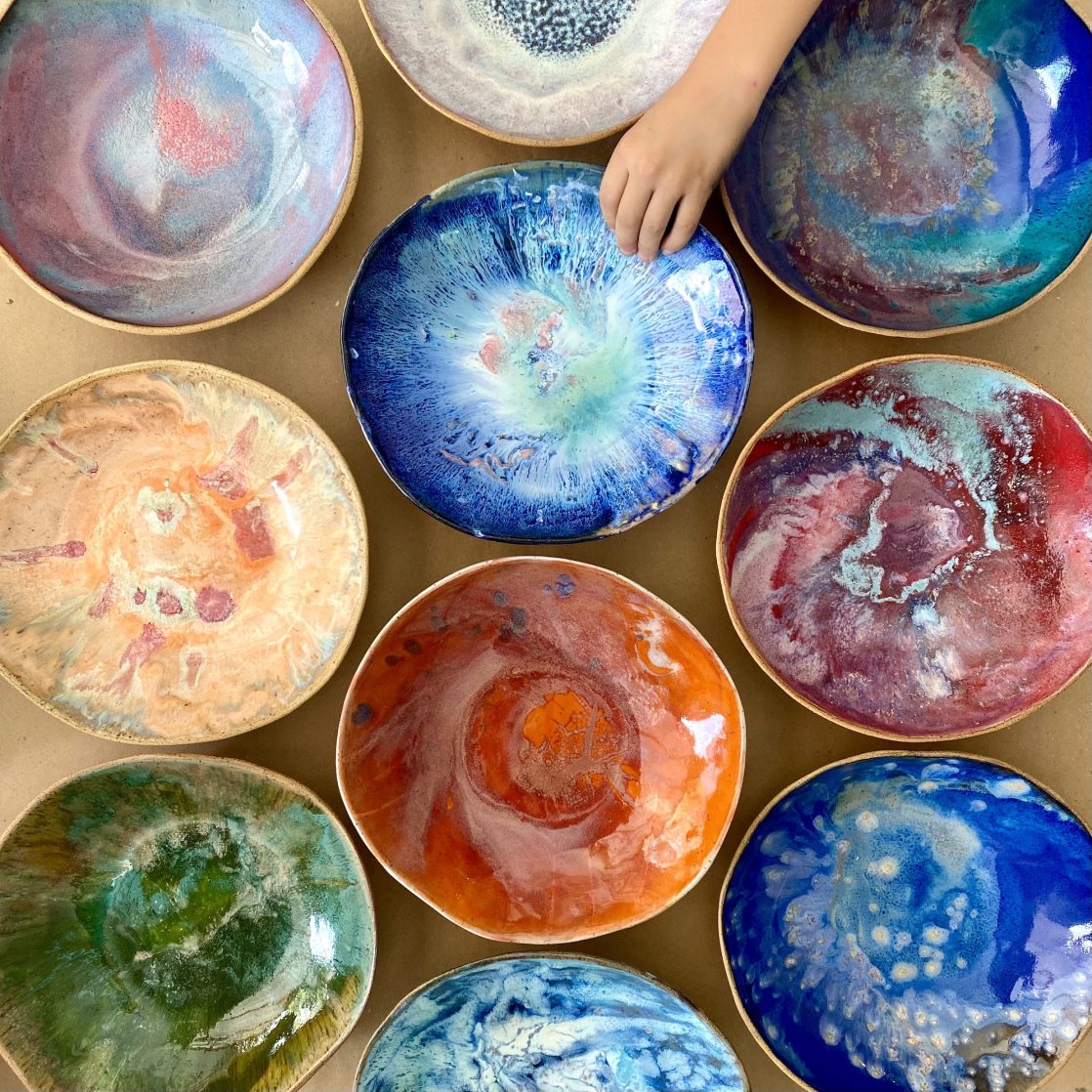A bright, detailed aerial photograph showcases an assortment of 10 handmade ceramic bowls displayed on a brown wrapping paper background. These bowls, each uniquely glazed, exhibit an array of stunning colors and patterns. Dominated by hues of blue, the collection includes four bluish bowls: one vivid cobalt blue, one blue and reddish-pink with a cosmic explosion effect, one marbled blue that looks like the earth from space, and another with various blue tones. Other vibrant bowls in the mix are a striking red, a bright orange, a green, a peach with ochre accents, and a couple predominantly white with speckled mixed colors. The bowls feature mottled and marbled glazes with some even rimmed in gold, adding to their artisanal beauty. Attention is drawn to a left hand, likely of a child, appearing in the upper right corner, gently touching one of the cobalt blue bowls. The bowls are arrayed with four centrally placed and three on either side, with a few only partially visible.